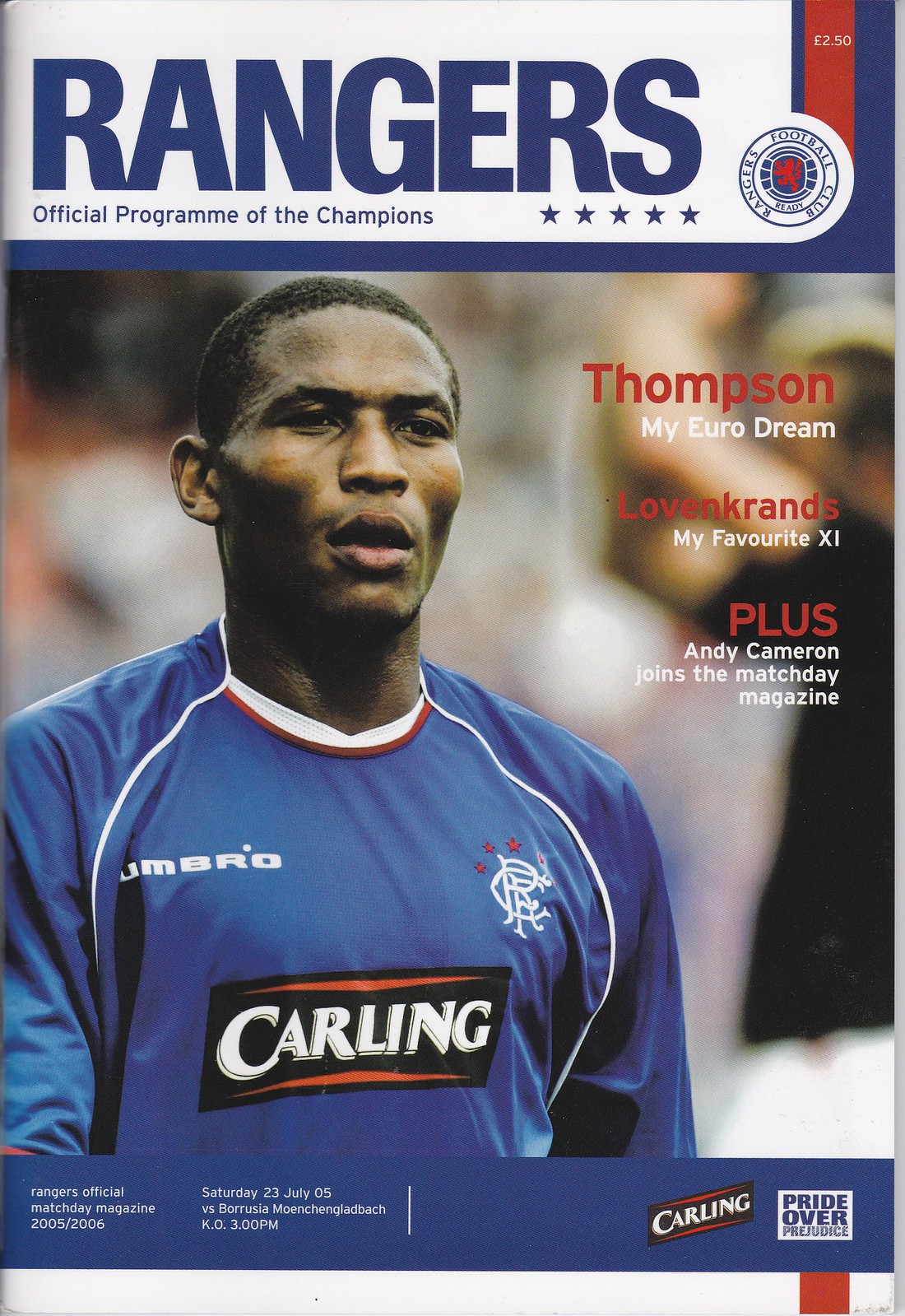The cover of the 2005-2006 Rangers official match day program prominently features an African American player from the soccer team, wearing a blue and white jersey with "Carling" and "Umbro" logos. Above the player, in large dark blue letters on a white background, it says "Rangers," followed by "official program of the champions" in smaller text, alongside five stars. The main headline, "Thompson, My Euro Dream," is written in bold letters with "Thompson" in red. Additional article titles include "Loving Crayons: My Favorite 11," and "Plus: Andy Cameron Joins the Match Day Magazine," with key words like "Loving Crayons" and "Plus" highlighted in red.

A red bar across the top mentions a price of "2.5 Euro." Below the player, a blue bar reads "Rangers Official Match Day Magazine, 2005-2006, Saturday, 23rd July 05, versus Borussia Mönchengladbach, kickoff 3 p.m." In the bottom right corner, two sponsor logos, "Carling" and "Pride Over Prejudice," are displayed. The background is blurred, emphasizing the player’s focused gaze into the distance, and the overall design directs attention to the cover's main elements.